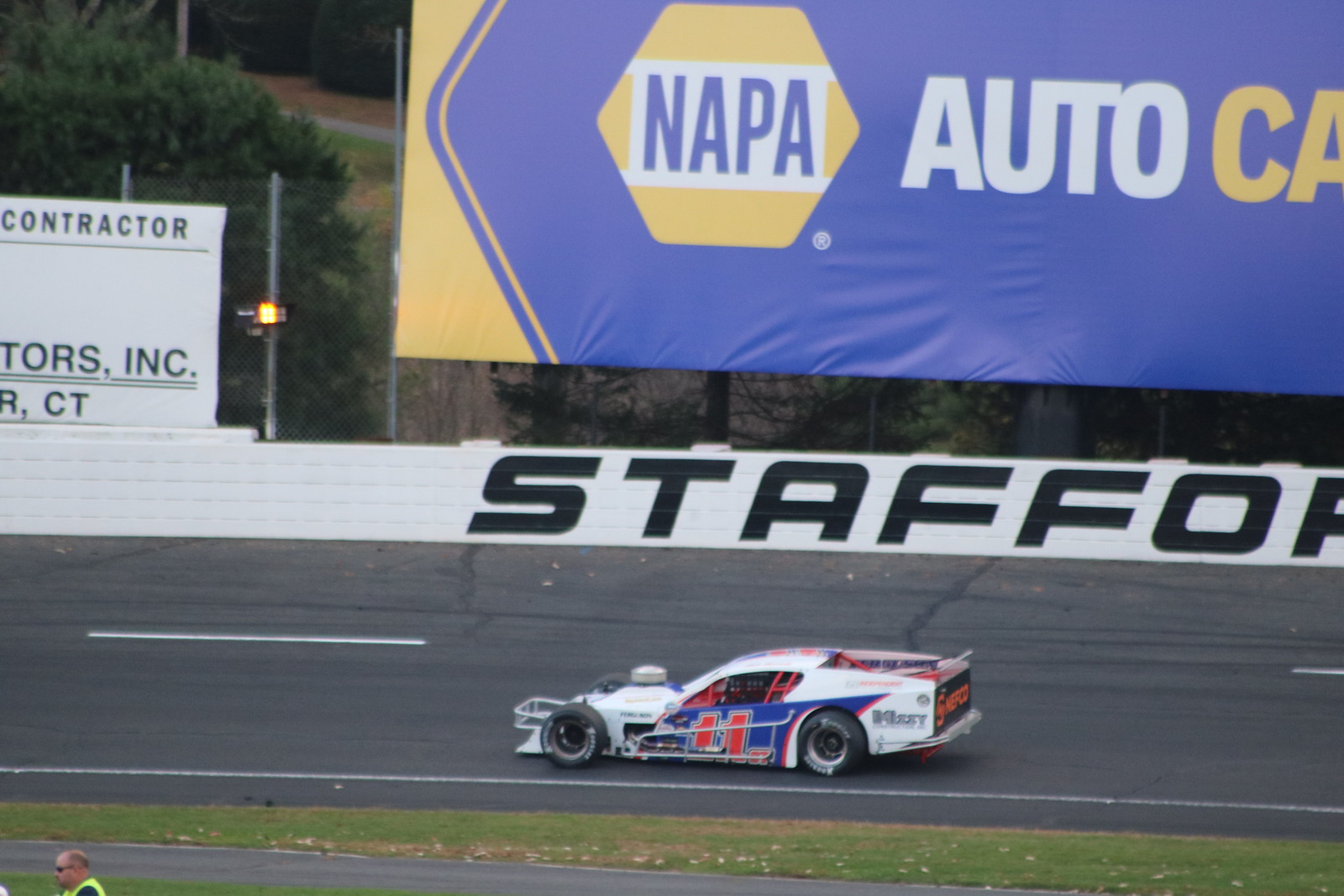This image captures a bustling daytime scene at an outdoor racetrack. The focus of the image is a white racing car adorned with blue decals and the red number 11, accentuated by its wide Hoosier tires, as it speeds towards the left on an asphalt track with crisp white markings. A man wearing sunglasses and a neon green emergency vest stands on the bottom-left corner near a small strip of grass. The track is enveloped by a white retaining wall with segments of black letters spelling out "STAFF," partially obscured by the barricade. To the right, a prominent blue and yellow sign for "NAPA AUTO CARE" towers above the wall, accompanied by another white sign that reads "CONTRACTOR." The far side of the racetrack curves upward, likely indicating the entrance or exit of a turn, while trees and wooded areas are visible in the distant background.